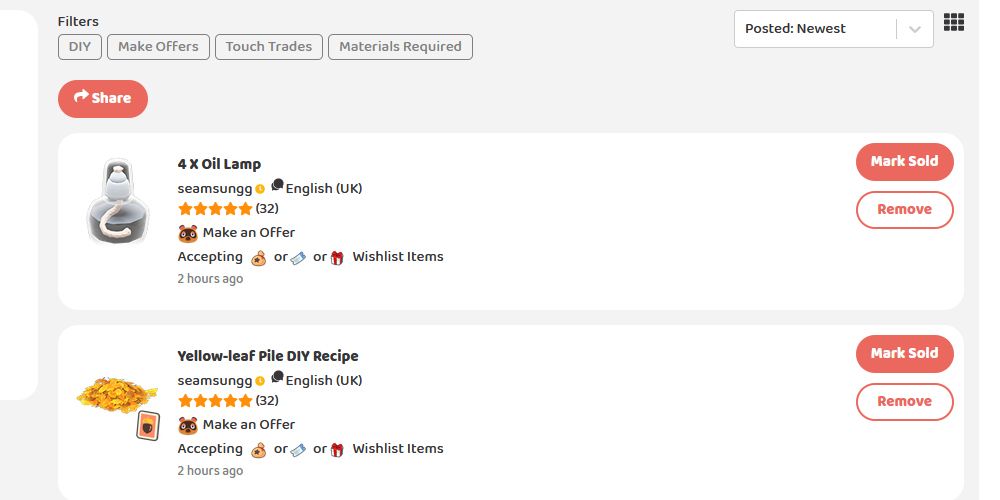A detailed caption for the described image:

The image showcases a section of a unique online shopping interface with a predominantly white background and subtle light grey dividers. At the top, there are rectangular filters labeled "DIY," "Make Offers," "Touch Trades," and "Materials Required," all bordered in black with light grey text. A dropdown menu with the selection "Product post: newest" is situated on the right side, next to a small square icon featuring three rows of tiny black squares. On the left, a curved red "Share" button, with the word "Share" in white, is prominently displayed.

The first product listed is titled "4x Oil Lamp - Samsung" with a UK English description, boasting a five-star rating from 32 reviews. It offers the option to "Make an offer," indicated by an icon resembling a bag of money. The listing was posted two hours ago. Accompanying the text is an image depicting two grey circles stacked vertically with a white cord trailing from the bottom. To the right of the image are two buttons: a red "Mark Sold" button with white text and a white "Remove" button with red text.

The second item is a "Yellow Leaf Pile - DIY Recipe," also by the same seller with identical ratings and offer options. The description suggests it's part of a DIY project involving yellow leaves, although the accompanying small square icon between the listings is ambiguous. Similar to the first item, this listing includes "Mark Sold" and "Remove" buttons.